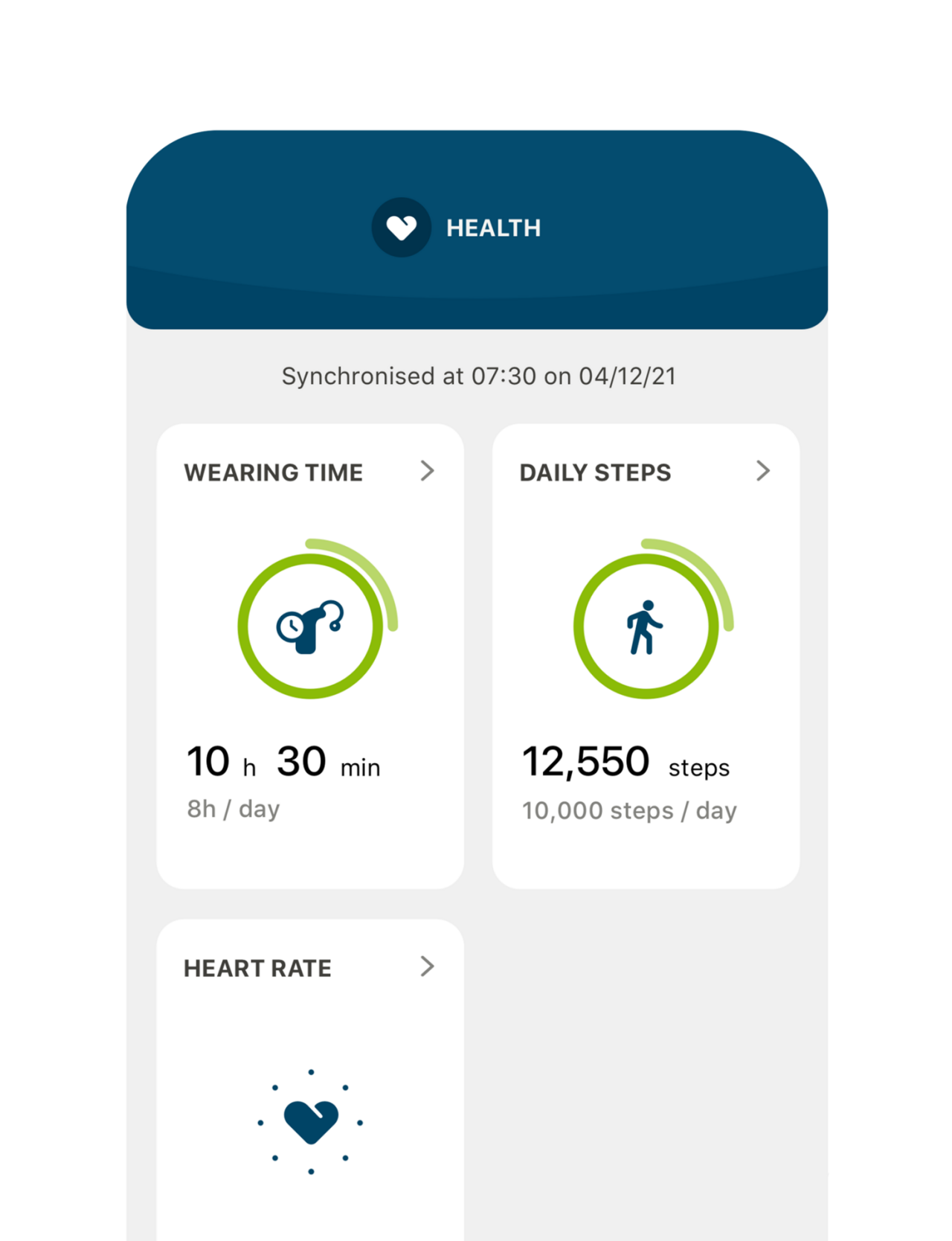The image is a screenshot from a phone app with a predominantly gray background. At the top, there is a light bluish-green label featuring a white heart icon followed by the word "health" in white text. Directly beneath this, black text reads "synchronized at 7:30 on 4-12-21." Below, there are three distinct white boxes, each presenting different health metrics. The first box displays "wearing time" and indicates "10 hours, 30 minutes," with additional text noting "8 hours a day" and a circular icon resembling a clock. The second box represents "daily steps," listing "12,550 steps" and highlighting a goal of "10,000 steps a day," accompanied by an orange icon depicting a person walking encircled by dots. The third box is labeled "heart rate," featuring a blue heart icon encircled by blue dots, but no heart rate information is visible.